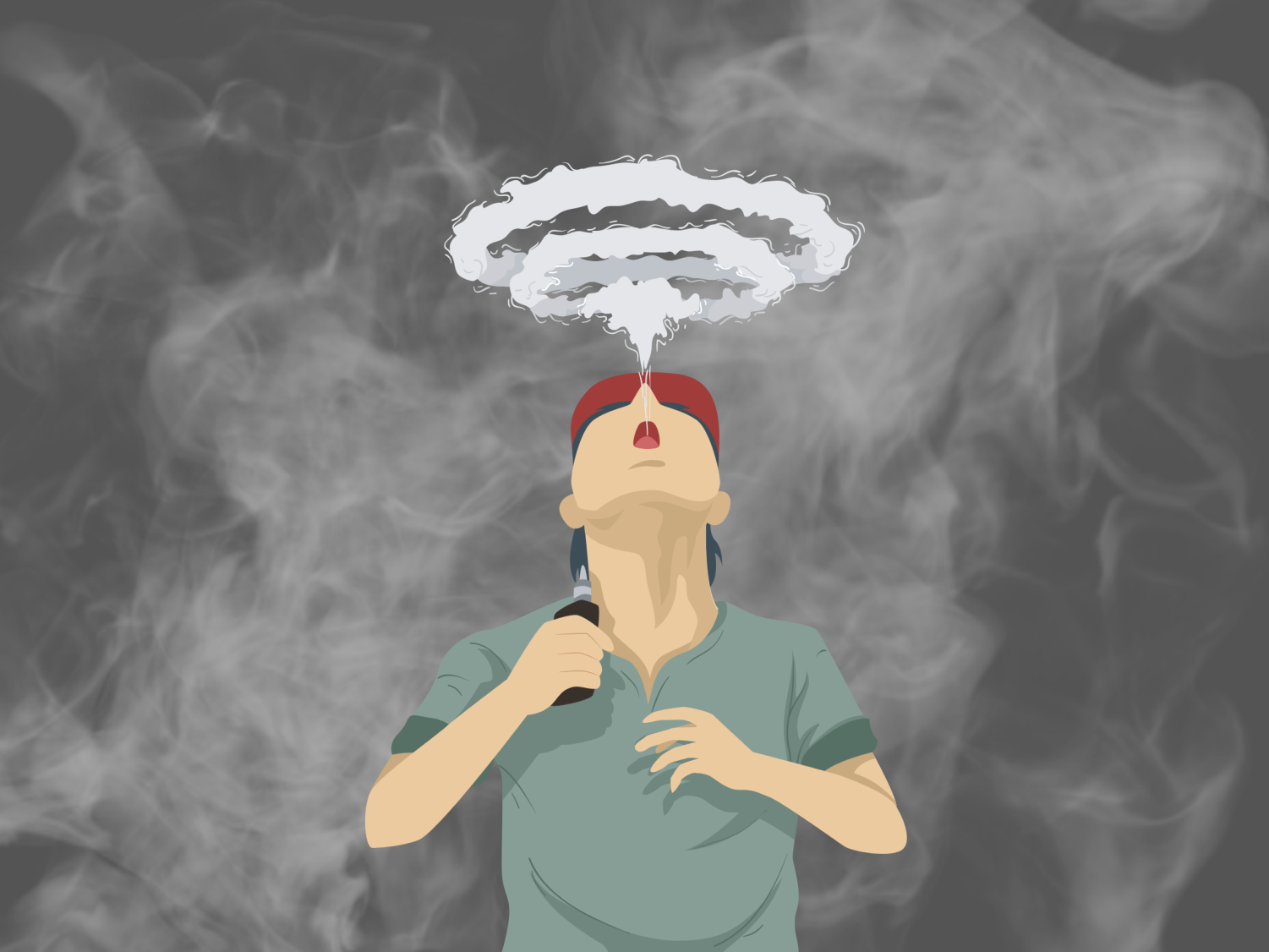This digital drawing, resembling a comic book illustration, features a person, likely a man, wearing a red baseball cap and a light green shirt with dark green sleeves. Positioned centrally, his head is tilted back, mouth open, and nose pointed upwards, blowing smoke rings into the air. His right hand holds a vape pen with a black body and white tip, while his left hand is closer to his chest. The background stands out with its realistic smoke effects against a black backdrop, creating a stark contrast between the digital art and the lifelike smoke. The overall color palette includes light green, dark green, red, black, gray, white, and tan, enhancing the vividness and depth of the scene.